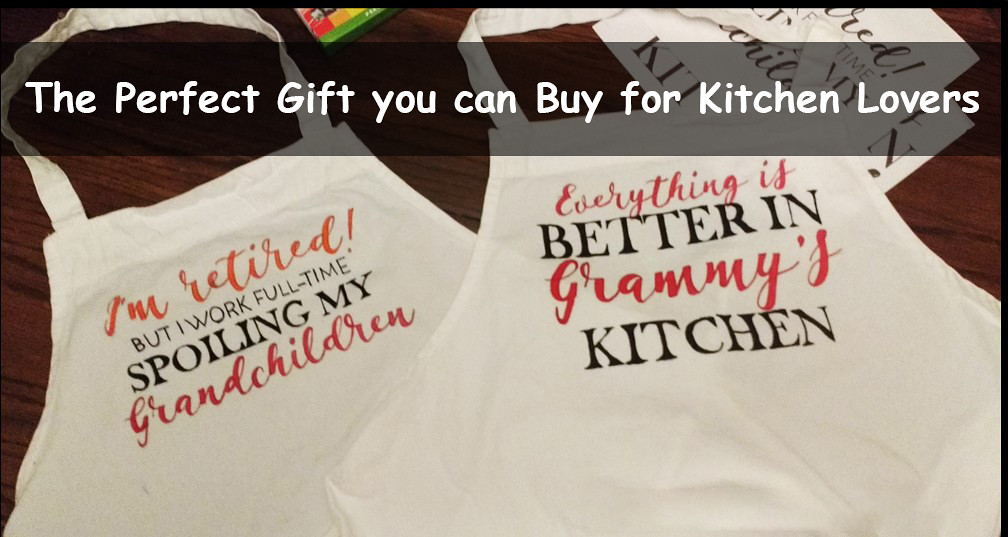This photograph features two aprons lying flat on a wooden surface. The apron on the right reads, "Everything is better in Granny's kitchen," with the words "Everything is" and "Granny's" written in red cursive, while "better in" and "kitchen" are in black print. The apron on the left states, "I'm retired but I work full time spoiling my grandchildren," where "I'm retired" is in orange cursive, "but I work full time spoiling my" is in black print, and "grandchildren" is in red cursive. Both aprons are white and designed to go around the neck, not just tie at the waist. The scene also includes a transparent grey or black box with white text that says, "The perfect gift you can buy for kitchen lovers," and there's a small green object at the top of the image.